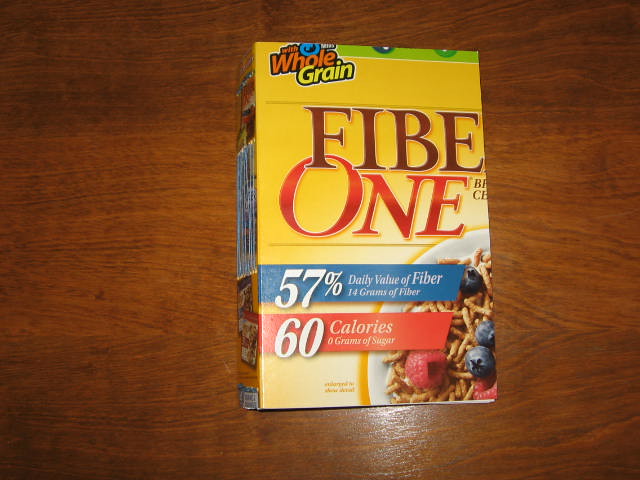This photograph depicts a yellow Fiber One cereal box lying on a medium dark brown wooden table. The front of the box, slightly cut off, displays "F-I-B-E" with "1" directly below in bold red letters, indicating "Fiber One." The visible side of the box features important nutritional information, including a prominent 57% daily value of fiber, equating to 14 grams, and highlights of 60 calories and 0 grams of sugar. The cereal box also boasts it is made with whole grain, noted by a symbol in the top left corner. The box background includes a vibrant image of the cereal, showcased in a white bowl topped with raspberries and blueberries. The image quality suggests the box might be slightly aged, and the lighting, while fair, reveals additional but unreadable writing along the side and bottom.